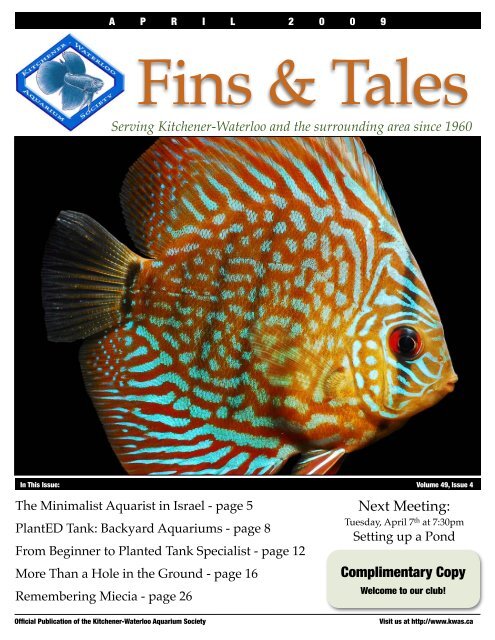The cover image is of a periodical called "Fins and Tails," serving Kitchener, Waterloo, and the surrounding area since 1960. Featured prominently in the center is a stunning angelfish with a golden body adorned with intricate turquoise and neon blue accents. The fish’s tail fans out in a semi-transparent quality, edged with the same vibrant hues that highlight the dorsal and ventral fins. The angelfish’s large, expressive eye is a striking mix of black and red, complementing its overall vivid appearance.

The header of the magazine includes "April 2009" and the title "Fins and Tails" written in orange. Additionally, a logo of the Aquarium Society of Kitchener-Waterloo, colored in blue, is displayed on the upper left corner. The text notes that this is a complimentary copy and welcomes readers to the club, mentioning the next meeting scheduled for Tuesday, April 7th at 7:30 p.m., focusing on pond setup.

The periodical promises a variety of engaging articles, including "The Minimalist Aquarist in Israel" on page 5, "Plants, Earth, Sand, Backyard Aquariums" on page 8, "From Beginner to Planted Tank Specialist" on page 12, and "More Than a Hole in the Ground" on page 16. It’s clear this publication caters to aquarium enthusiasts with a rich array of content.